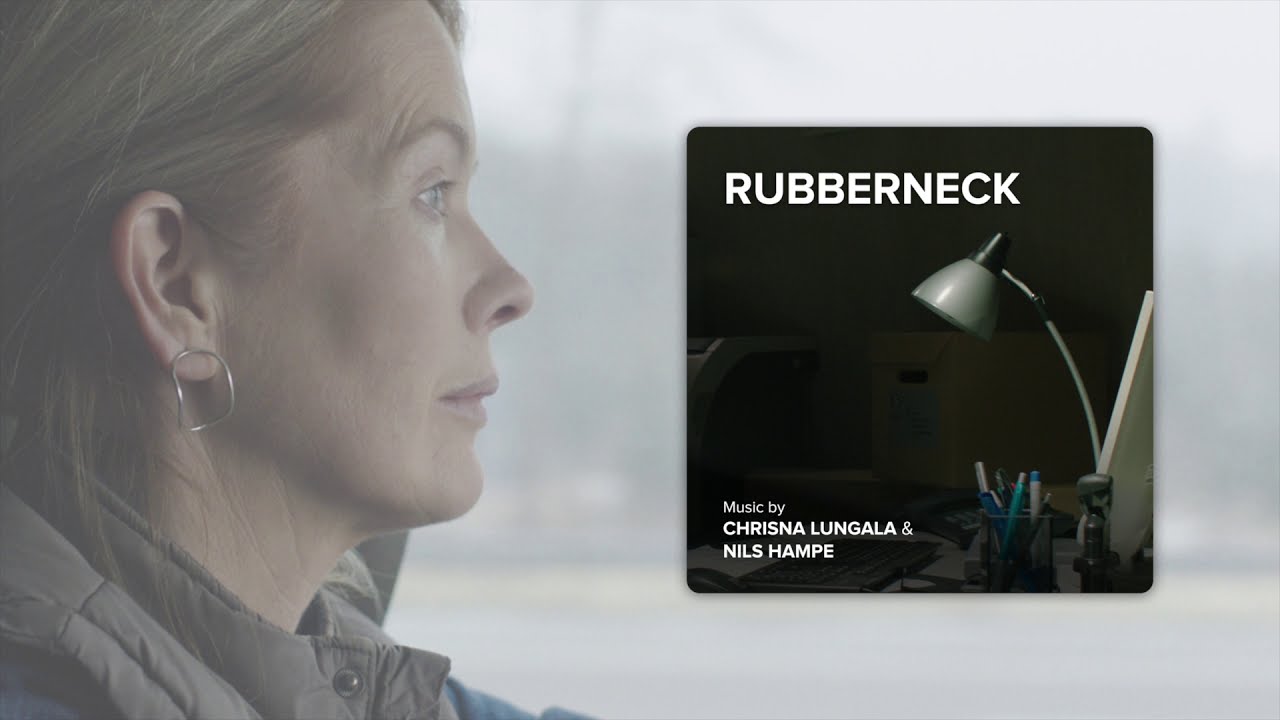This image features a white woman, likely in her 50s, who is gazing intently to the right, perhaps out a window or windshield, suggesting she might be in a car. She has long, blondish-brown hair with some gray, and is wearing a brown vest over a blue long-sleeved shirt. Her right ear is adorned with a circular earring that is slightly oblong. The photo is somewhat hazy and dark, indicating low lighting conditions.

On the right side of the image, there's a prominently displayed black square with a white font that reads "Rubberneck" at the top, and "Music by Krishna Lungala and Nils Hamp" at the bottom. This area features elements that suggest it's an album cover, including a work desk with a silver arched desk lamp (which is turned off), a flat screen computer, a keyboard, sticky notes, and a container with pens. The background of this section appears mostly black, contrasting the woman’s setting and providing an artistic cover feel. The juxtaposition of the lady in a thoughtful pose and the detailed elements of the desk setup hint at a blend of introspection and creativity, likely representing themes of the album or CD.